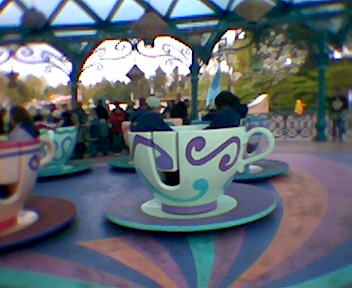This photograph captures a colorful teacup ride, likely at Disneyland or a similar amusement park. The ride features a vibrant floor painted with swirling patterns in shades of green, pink, blue, and orange. Five teacups, each painted with distinctive swirling designs, are arranged on the floor, with each teacup accommodating two people. The teacups prominently display intricate color schemes, with the most visible one being teal with teal and purple swirls. Another teacup, mainly pink with purple and darker pink swirls, adds to the vivid display. The canopy over the ride appears to be glass supported by green poles, allowing natural light to filter through. In the background, the iconic Disneyland towers and some greenery can be glimpsed, enhancing the whimsical atmosphere of the scene.